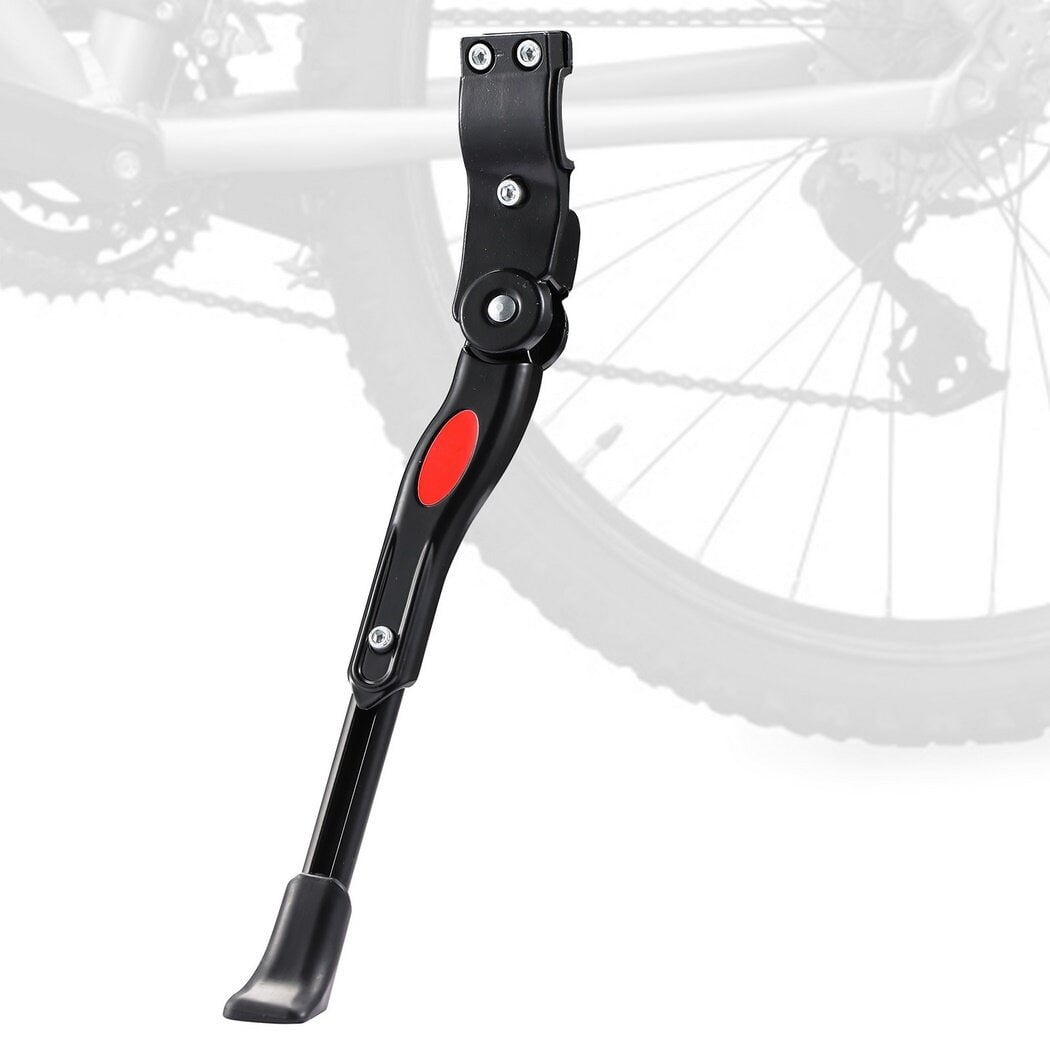This detailed product photograph showcases an attachable and detachable kickstand designed for a bicycle. The kickstand, primarily black in color, features a small red oval in the center, presumably for branding purposes. It attaches to the back side of the bicycle via three silver rivets and includes a hinge joint, allowing it to be positioned upwards when the bike is in use and downwards to support the bike. The end of the kickstand, which touches the ground, has a black tip resembling a boot. In the background, a faint and less detailed image of a bicycle is visible, including the chain, wheels, tires, and the valve stem for inflating the inner tube. The bike frame itself appears grayish and serves to illustrate the correct position of the kickstand on the bicycle.